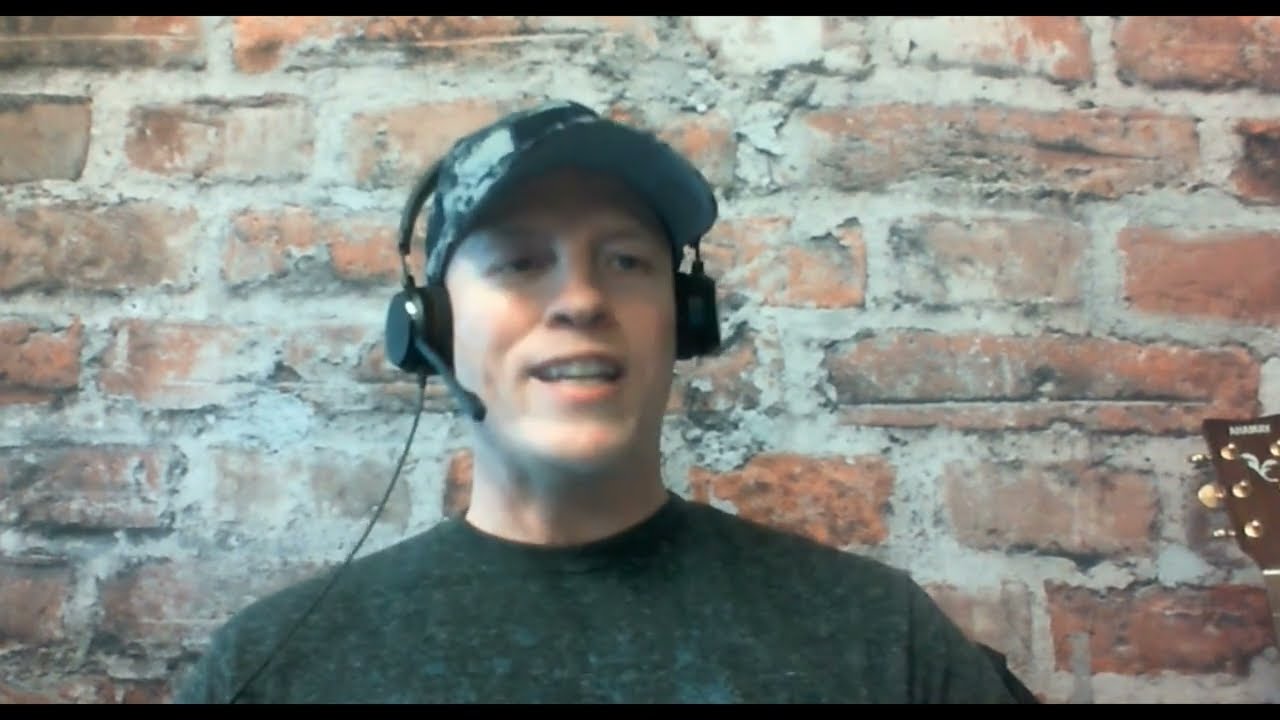The image depicts a close-up view of a white man seated with a black and white baseball cap on his head. He is sporting a black headset with a boom microphone that extends to his mouth, which is slightly open as if he is talking or smiling. A wire hangs down from the headset. The man is wearing a forest green, long-sleeved shirt with a subtle white speckling pattern. To the right of the man, the neck and tuning knobs of a dark brown wooden guitar with golden adjustment parts are visible, leaning against the wall.

The background showcases a large, horizontally laid brick wall with reddish-brown bricks and uneven, aged gray mortar between them. The wall extends across the width of the image, which is a wide rectangular frame. Thin black strips border the top and bottom of the photo. The man is positioned centrally and is visible from the shoulders up, looking slightly to the right.